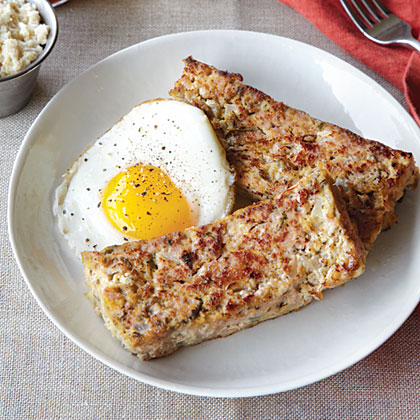The image features a white plate resting on a gray tablecloth, showcasing a breakfast dish. At the center of the plate are two rectangular, browned pieces of food, which might resemble either a type of breakfast pizza, French toast, or another toasted bread item. Next to these pieces, there's a sunny-side up egg with a bright yellow yolk and scattered black pepper. In the background to the upper right, a metal fork is placed beside a red napkin. Additionally, at the top left of the image, there is a small bowl containing a white condiment or another side dish.